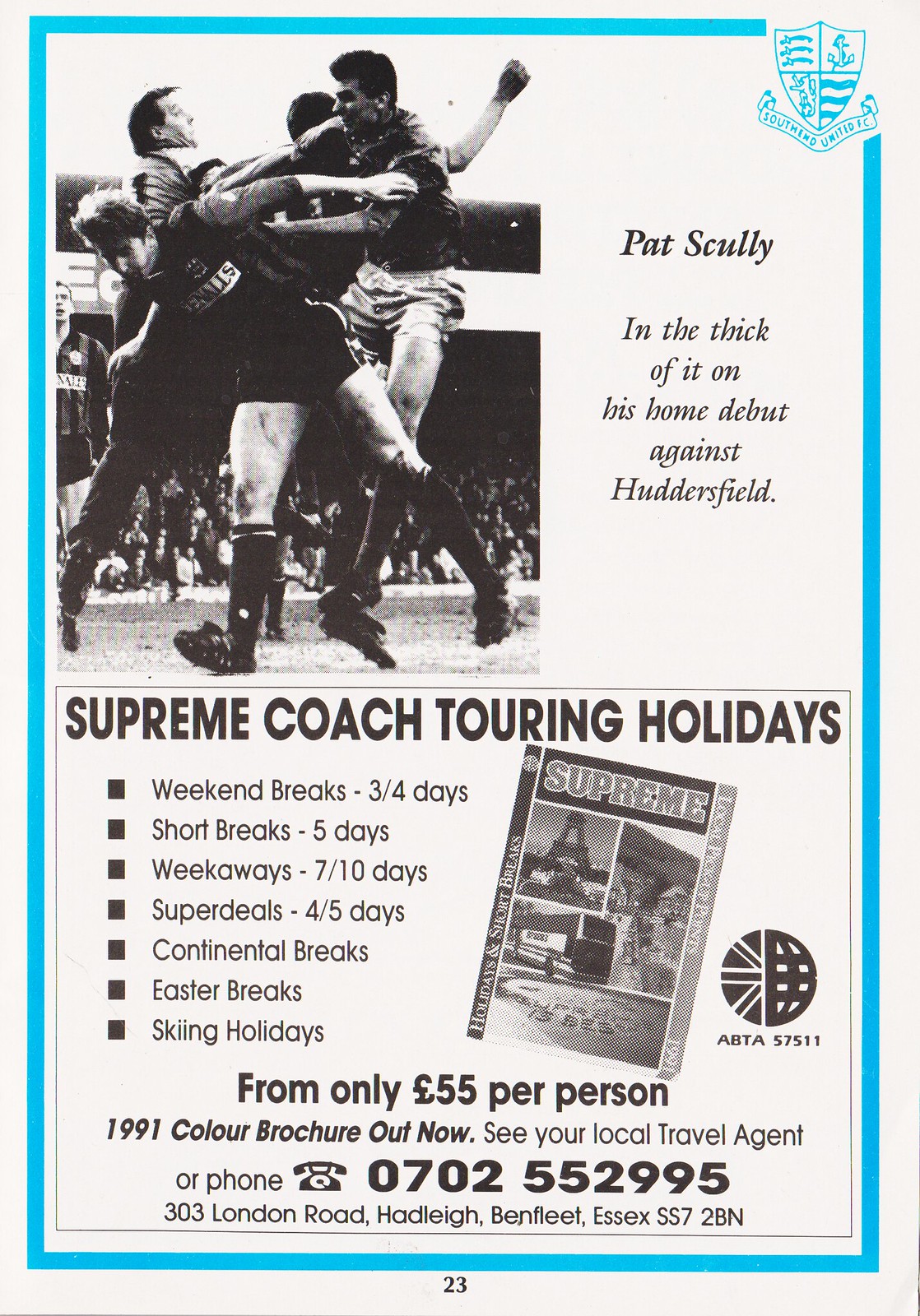This image appears to be a page from an old sports magazine, characterized by its vintage aesthetic and a predominantly light blue, black, white, and various gray color palette. The main focus is a photograph in the upper left corner depicting several football players. The text accompanying the image reads, "Pat Scully in the thick of it on his home debut against Huddersfield." Below the photograph, there is an advertisement for "Supreme Coach Touring" which offers various holiday packages: weekend breaks (three out of four days), short breaks (five days), week-long trips (seven out of ten days), super deals (four out of five days), as well as specific options for continental breaks, Easter breaks, and skiing holidays. The single sheet largely occupies the entire frame, further emphasizing that the image is of a magazine or book page, notable for its nostalgic and retro design.